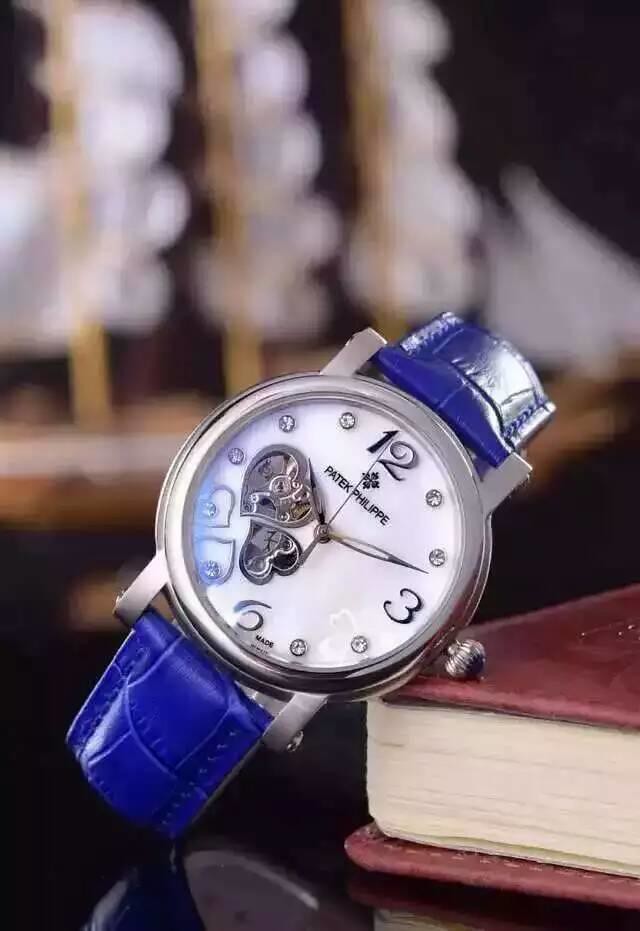This is a close-up portrait-mode photograph of a very expensive Patek Philippe wristwatch, expertly showcasing its luxurious design. The watch, characterized by its brushed silver or possibly stainless steel body, features a meticulously crafted white face with a pearlescent sheen. Key indices at 12, 3, and 6 are marked in black, while the remaining hour indices at 1, 2, 4, 5, 7, 8, 9, 10, and 11 are adorned with diamonds, excluding the number 9 position which is replaced by two intricately cut heart-shaped cutouts. These open hearts provide a captivating view of the internal mechanisms and gears of the watch, adding a unique complexity to its aesthetic.

The watch is indicating the time as 10:12, with its metal hour, minute, and second hands pointing precisely. Below the 12 o'clock position, the brand name "Patek Philippe" is elegantly inscribed in black capital letters, along with a small four-leaf clover-like emblem positioned between the "12" and the brand name.

The timepiece is secured with a striking bright blue faux alligator leather strap, which stands out vividly against the vintage leather-bound book it leans upon for support. The watch is angled to rest its bezel, skillfully crafted in brushed silver, against the edge of the book, with its bottom strap touchingly gently the surface below. The background features a blurred artistic rendition of white trees, contributing to an overall serene and sophisticated ambiance, enhanced further by the slight shadow cast on the foreground, possibly by the strap. Additionally, an out-of-focus wooden model ship can be seen, adding a touch of classic decor to the scene.

Every element in the photograph works harmoniously to emphasize the elegance and craftsmanship of this Patek Philippe watch, from the gleaming diamonds and intricate heart cutouts to the rich blue leather strap and the blurred, sophisticated background.